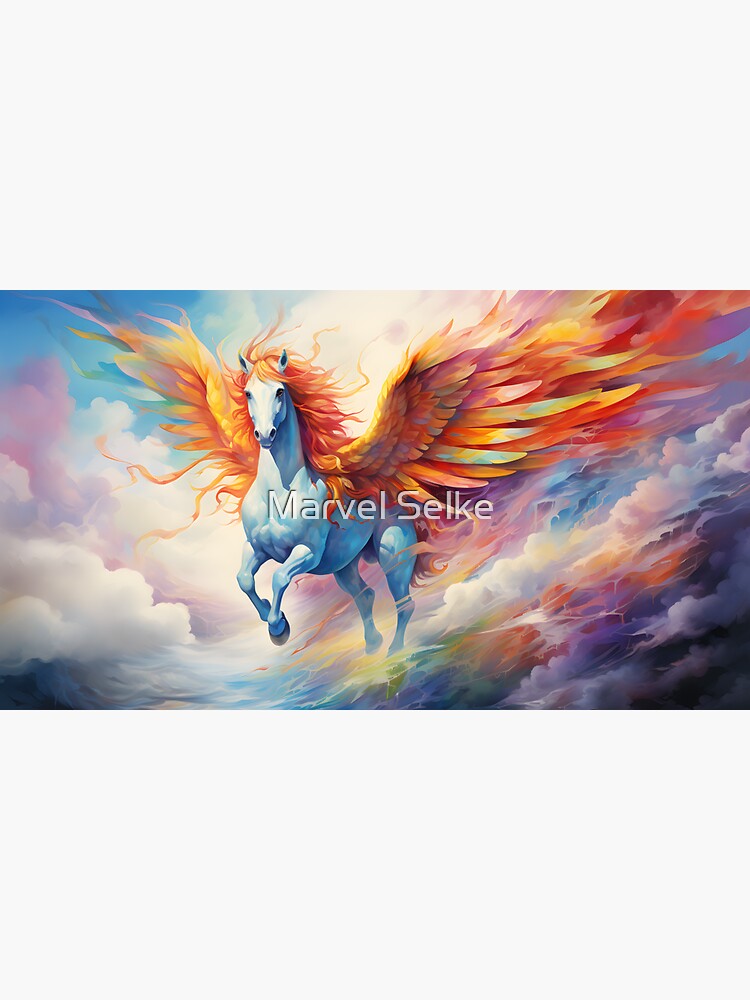The image depicts a vibrant and fantastical Pegasus flying through the sky, its body a pure, brilliant white. The Pegasus is adorned with large, elaborate wings displaying a swirling palette of rainbow colors, predominantly fiery orange. Its flowing mane, swept back by the wind, radiates in shades of orange, with hints of pink and red adding to the ethereal quality of the scene. The creature soars amidst a dreamy backdrop of clouds, which are awash with primary colors strikingly vivid on the right-hand side and more subdued, featuring whites and soft pinks, on the left. High above, the blue sky and a bright, shining sun complete the majestic composition. A watermark reading “Marvel Selkie” is prominently displayed across the image, adding a touch of mystery and suggesting inspiration from Marvel's stylistic creations. This whimsical and detailed artwork presents a uniquely colorful and imaginative vision.